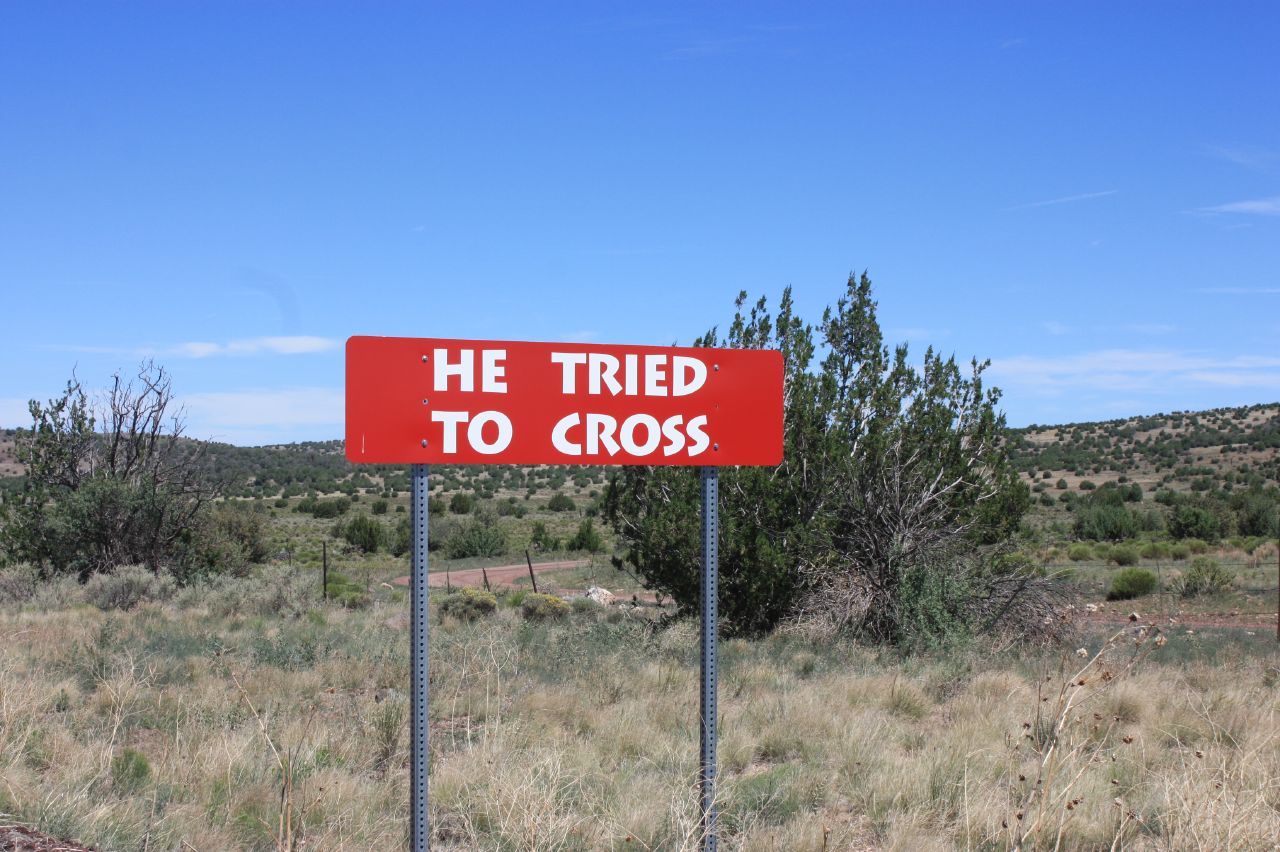The image captures a serene natural setting featuring a grassy field beneath a clear blue sky. Dominating the foreground is a red sign mounted on two silver perforated metal posts. The sign, bearing white text humorously proclaiming "He tried to cross," suggests a tongue-in-cheek alert, likely situated by the roadside. The field is a tapestry of various shades of green and brown, indicative of overgrown and slightly withered grass. A prominent, darker green bush stands in the middle, flanked by another on the left-hand side. As the eye moves towards the background, the field transitions into patches of brown and green grass interspersed with an assortment of bushes in various sizes and darker hues of green, adding depth to the landscape.